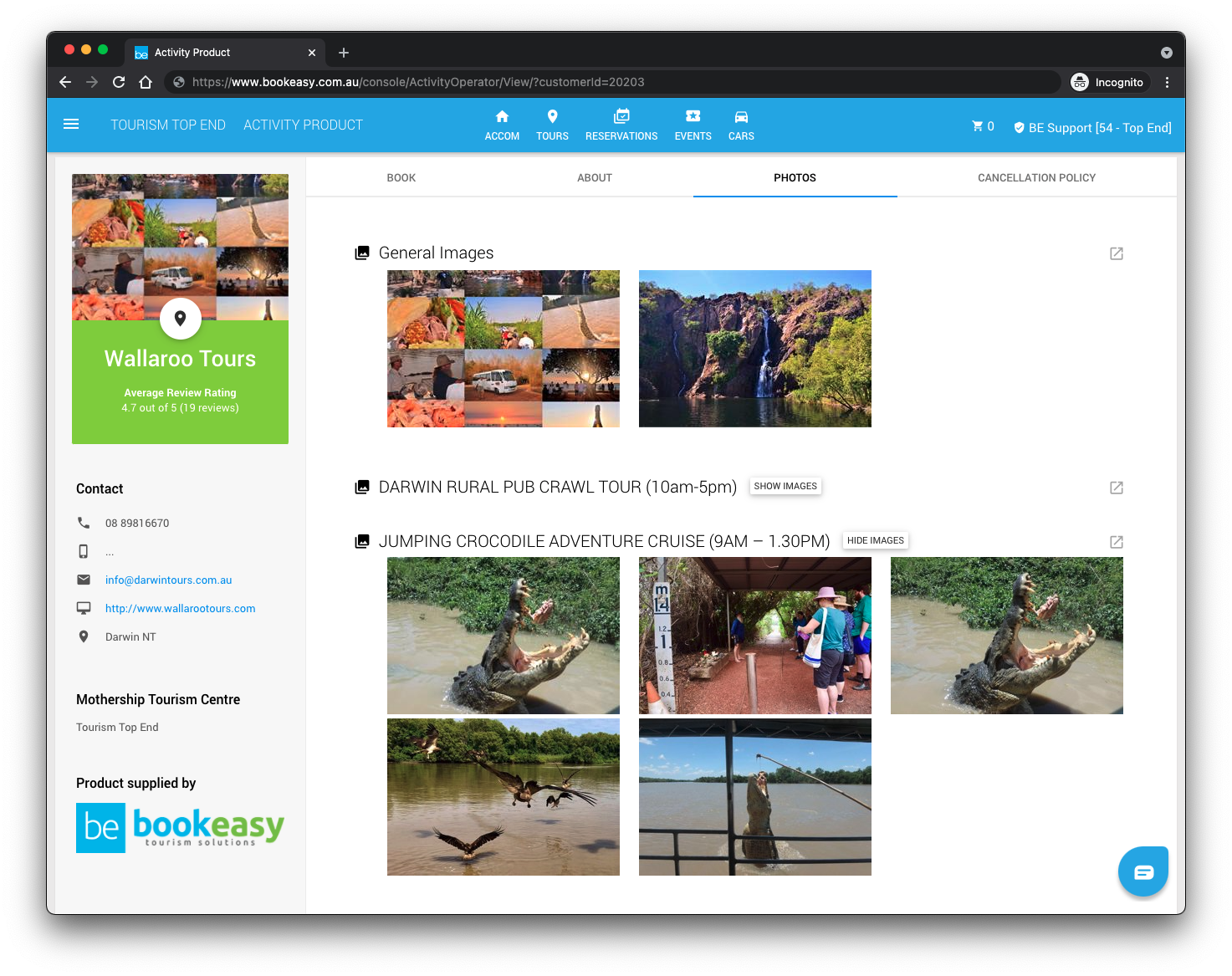The screenshot captures a webpage open in a web browser with a single tab titled "Activity Product" visible. The URL displayed in the address bar reads "bookeasy.com.au/console/activityoperator/view/?customerID=20203". The browser is in incognito mode as indicated by the icon and three vertically aligned dots in the upper right corner. Standard navigation buttons for back, forward, refresh, and home are present below the address bar.

A blue navigation strip runs across the top of the webpage containing a menu icon represented by three horizontal lines, followed by the text "Tourism Top End Activity Product". Centrally positioned are various menu options: "ACCOM", "Tours", "Reservations", "Events", and "Cars". On the far right, a shopping cart icon displays "0", next to "BE Support", with the text "(54-top end)".

Further down, the page displays information about "Wallaroo Tours", spelled "W-A-L-L-A-R-R-O-O Tours", featuring an average review rating of 4.7 out of 5 from 19 reviews. Contact information for the Wallaroo Tours is listed below. The site appears to be part of "Book Easy Tourism Solutions".